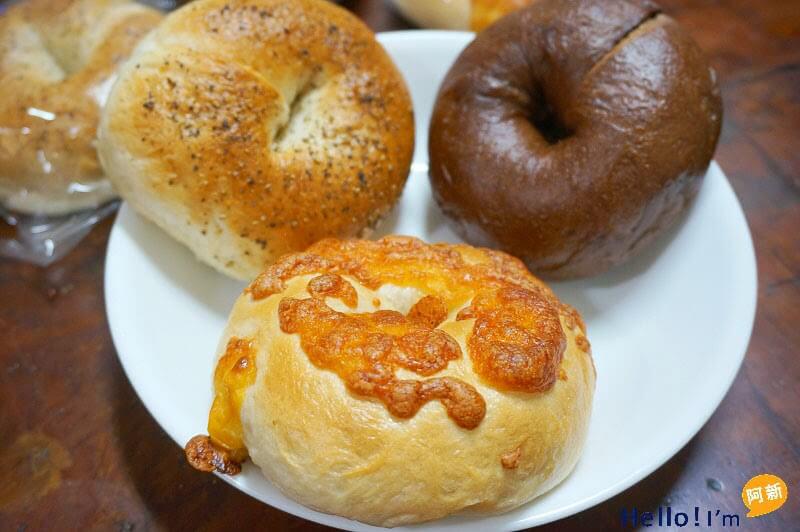In the center of the image, there is a white ceramic plate displaying three distinct bagels arranged clockwise. At the bottom middle, there is a bagel topped with melted, slightly orangey-brown Asiago cheese. Moving clockwise, the next bagel is lightly browned and covered with seeds, resembling an everything bagel. Beside it is a dark pumpernickel bagel, which has a small cut in its top right corner. In the top left corner, there is an additional bagel wrapped in a plastic bag, with the excess plastic gathered at one end. The scene is set on a dark wooden table. In the bottom right corner of the image, there is a greeting in black letters that reads "Hello!" followed by "I'm" and a speech bubble with an orange background, containing two non-English (Chinese) characters.